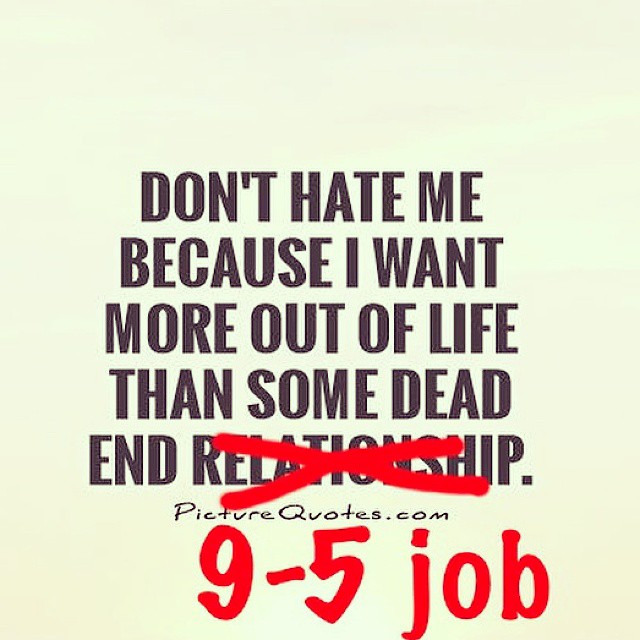This is an image of a vertical rectangular poster featuring a motivational message. The background is a greenish, light gray shade, and the text is centered in bold, black capital letters. Starting about a third of the way down from the top, the prominent message reads: "DON'T HATE ME BECAUSE I WANT MORE OUT OF LIFE THAN SOME DEAD END RELATIONSHIP." The word "RELATIONSHIP" is crossed out with a thick, red X, and underneath it is replaced with "9 TO 5 JOB" written in red paint. At the bottom, the source "picturequotes.com" appears in a handwritten-style script, with capitalized 'P' and 'Q'. The overall layout and design give it a striking and rebellious feel, emphasizing a desire for more fulfilling life choices.